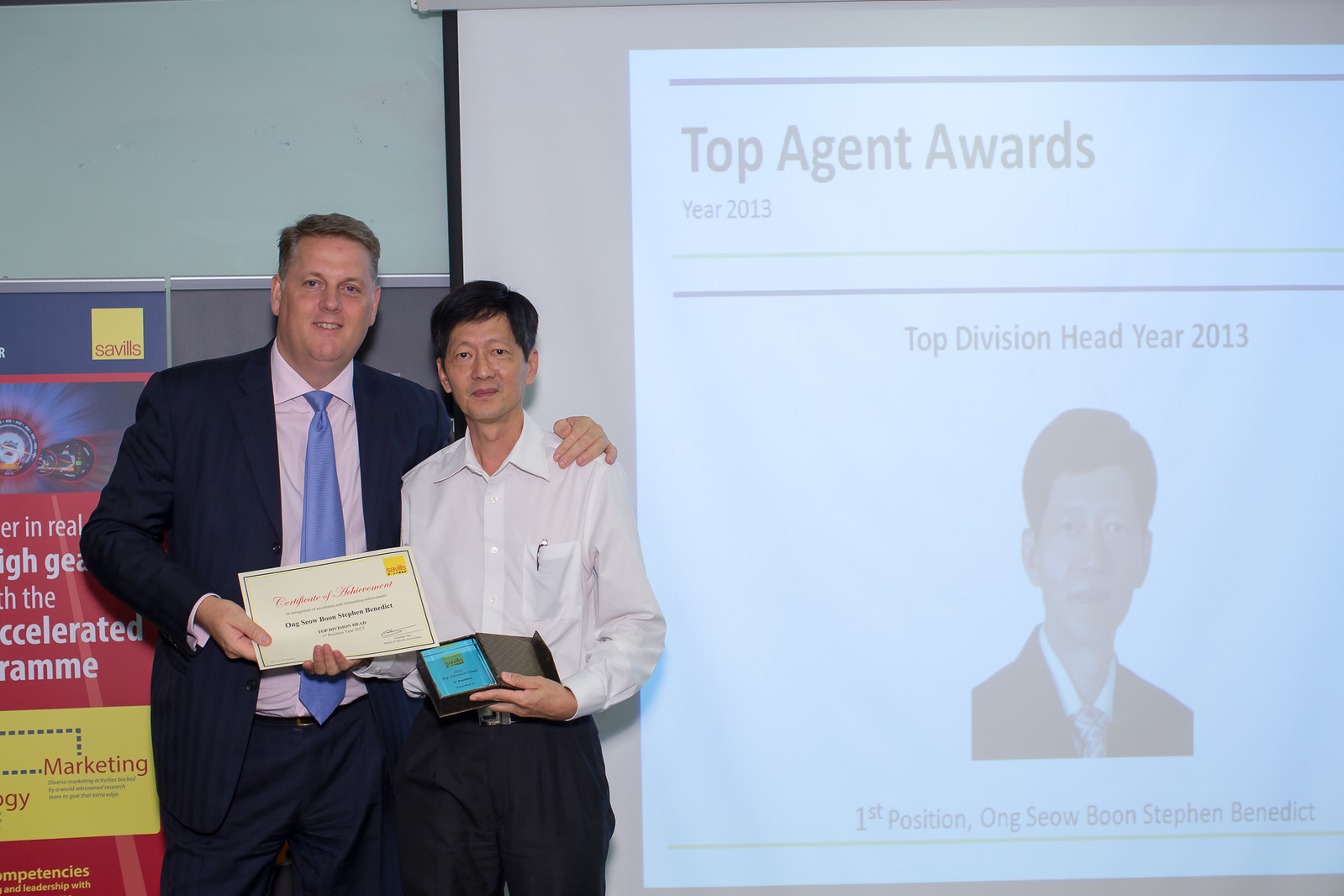In this photograph, two men are prominently featured in what appears to be an award ceremony. On the left side of the image stands an Asian man, likely in his early 50s, who closely resembles the individual shown in a projection on a nearby screen. This screen reads, "Top Agent Awards Year 2013," and "Top Division Head Year 2013," and prominently displays a black-and-white photo of the Asian man's head and upper body. The text on the projection also declares, "First Position Ong Siu Boon Stephen Benedict."

The Asian man is wearing a white dress shirt paired with gray slacks and is holding an award certificate in his right hand. In his left hand, he clutches what appears to be a book or plaque with a blue cover. Standing next to him is a slightly taller man of European or American descent, also seemingly in his early 50s. This gentleman is dressed in a gray suit, pink shirt, and blue tie. He has his left hand placed gently on the shoulder of the award recipient and is using his right hand to present the certificate.

Both men are smiling, with the presenter showing a broader smile. In the background, behind the two men, is a marketing poster, indicating their professional environment likely involves marketing. The setting clearly underscores the significance of the moment, celebrating the Asian man’s achievement as the top division head for the year 2013.